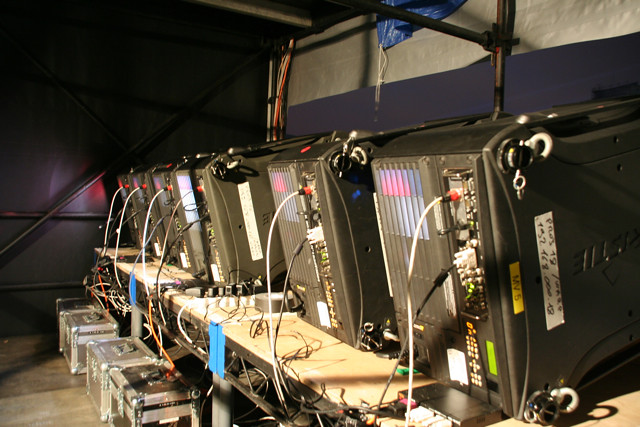The image depicts a row of six black electronic devices, possibly small furnaces or computers, aligned on light brown or tan tabletops in a dimly lit, unfinished basement setting. Each device has white electrical wires with red caps extending from the exposed electrical motor boards at the back of the equipment down beneath the tabletop. On the floor in front of each device, there are old-fashioned metal trunks or chests for storage. The room features exposed piping along the ceiling and has dark blue walls, adding to the industrial atmosphere. Various connectors are visible at the back of the equipment, contributing to the intricate and technical aesthetic of the scene.